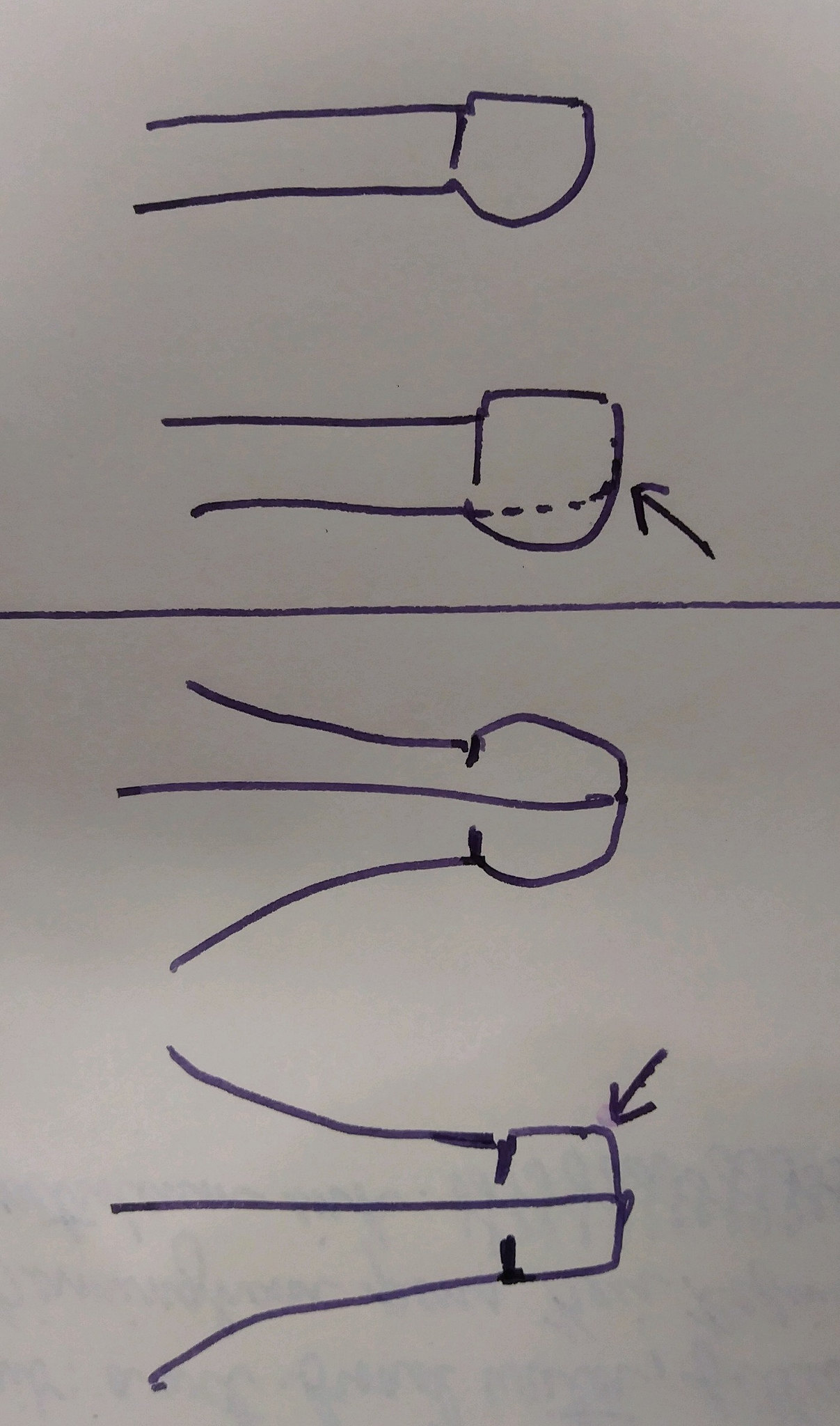The image depicts a minimalistic drawing on a textured gray paper that transitions from a lighter gray at the bottom to a darker shade at the top. The composition features five sequential knob-like structures. Each knob comprises two simple black vertical lines forming the stem and a rounded shape at the top, representing the knob itself.

From the top down:

1. The first knob is plain and unadorned, simply comprising two vertical lines and a round knob at the top.
2. The second knob mirrors the first but has an arrow pointing from the right side towards the left.
3. The third element, positioned just above a dotted line running horizontally across the middle, features a similar structure with an added horizontal line crossing its midsection.
4. Below the dotted line is another horizontal line spanning the width of the paper. Below this line, we find the fourth knob. This knob features two vertical lines, a central horizontal line intersecting the stem, and a rounded knob at the top.
5. The fifth and final knob, located at the bottom, displays a similar design to the fourth but includes an arrow at the upper right corner pointing downward.

This sequence of knob-like shapes with various lines and directional arrows provides a visual narrative that emphasizes simplicity and linear design elements.